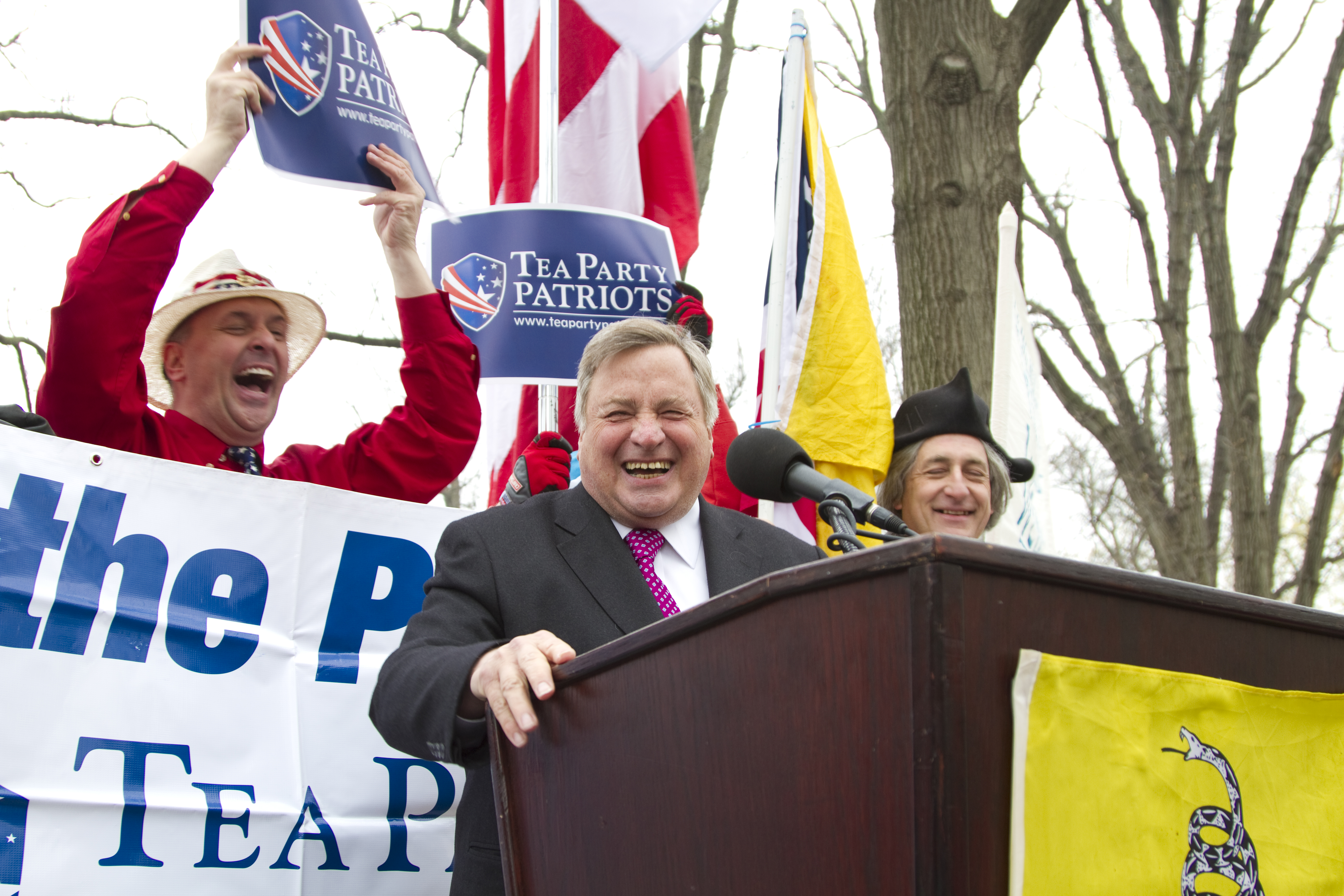In this photograph, a politician in his 50s or 60s stands at a large, brown wooden podium. He is smiling broadly and wears a gray suit paired with a white shirt and a magenta tie adorned with white polka dots. To his right, a man in a black hat reminiscent of the Revolutionary War era, with long gray hair, also smiles. Behind them, another supporter in a red long-sleeve shirt, blue tie, and a white brimmed hat holds a sign that reads "Tea Party Patriots," featuring a shield with red and white stripes and white stars on a blue background. The podium displays a yellow poster with a black and white snake, likely echoing the "Don't Tread on Me" symbol. In the background, flags with red and white stripes and other banners supporting the Tea Party are visible amidst barren trees, suggesting a fall or winter setting.